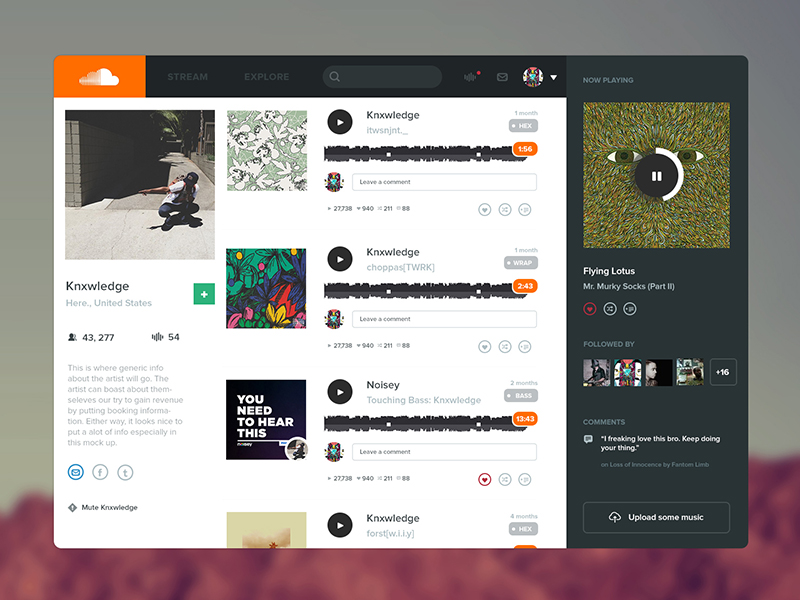The image depicts a vibrant web page interface, dominated by a central pop-up window against a gray and red background. The pop-up has an eye-catching orange background with a white cloud icon on the left. It features various navigation elements including a 'Stream' tab, an 'Explore' tab, a search bar, and an email option. Alongside these, a user profile icon, which is colored in blue, black, and red, is displayed in a circular frame with a heart button next to it.

In the main content area, there's a section titled "Now Playing" that showcases an album by Flying Lotus called "Mr. Murky Socks Part 3." The album cover is striking with its green and orange hues, adorned with two dark brown eyeballs. Below the album cover, user interaction options such as a heart button (enclosed in a red circle) and a shuffle button are available, along with a pause button for playback control.

At the bottom of the pop-up, a call-to-action invites users to "upload some music," highlighted by a cloud icon. Additionally, several other album covers are visible on the left side of the screen, suggesting a rich library of music available for exploration.